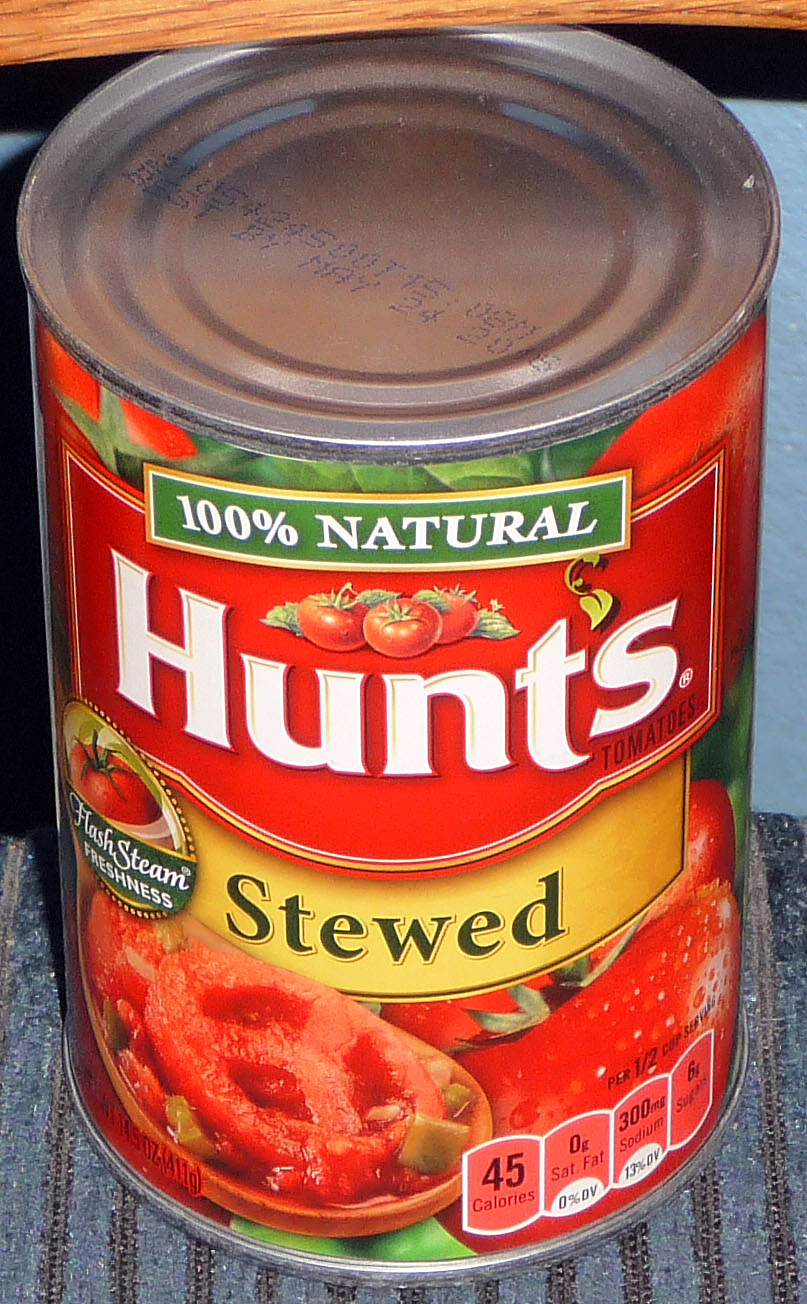This indoor digital photograph presents a close-up shot of a can of Hunt's stewed tomatoes in portrait mode. The can is prominently positioned in the center on a textured surface, likely a piece of gray carpet or an area rug, with darker gray stitching arranged in a grid pattern. To the sides of the image, a sliver of tan-colored wood with darker streaks is visible, contrasting with a predominantly blacked-out background on both the left and right sides.

The can's label is vividly detailed. At the top of the can, a green rectangle bordered in gold and white declares "100% Natural" in white lettering. Below this, a drawing of three red tomatoes with green leaves is displayed, followed by the brand name "Hunt's" in bold white letters on a larger red rectangle bordered in white. Underneath, a smaller yellow rectangle with dark green text reads "Stewed." To the left of this, a gold circle featuring another red tomato is crossed by a green banner with the cursive text "Flash Steamed," followed by the word "Freshness" in standard font beneath it. At the bottom of the label, a sliced tomato with some chunks alongside a whole tomato covered in water droplets is depicted. Additionally, nutritional information appears in black text within white-bordered rectangles, listing "45 calories," "0g sat fat," "300mg sodium," and "6g sugar" against an off-red background. The can also features a top label with blue print indicating "Best by May 24, 2016."